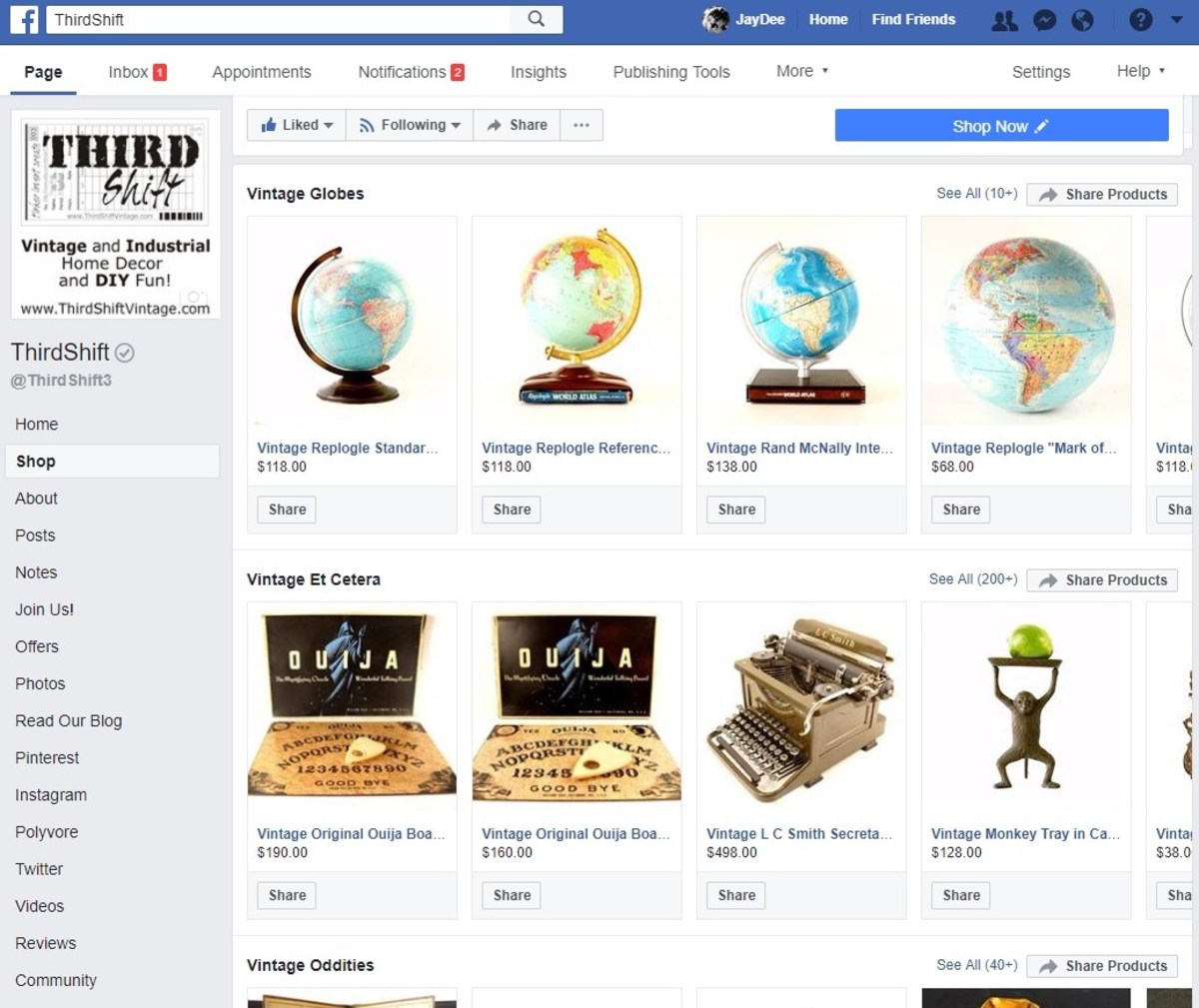The image depicts a screenshot of a Facebook page with a blue header. At the top left, there is a white square with a blue "F" representing the Facebook logo. Directly below, a white search bar contains the text "Third Ship" in black font, alongside a magnifying glass icon.

On the right side of the header, the menu displays "JD Home" and "Find Friends" in white text on a black background. Icons follow this text: two people (possibly representing friends or a group), another that might symbolize a messaging platform like Telegraph, a globe icon, a circle with a question mark, and a drop-down arrow.

The main content area of the page has a white background. Underlined in blue is a black-outlined page icon, followed by several menu options in black text: Inbox, Appointments, Notifications, Insights, Publishing Tools, and More. More white space leads to sections labeled Settings and Help.

On the left sidebar, there is a list of navigation options under "Third Shift," including Home, Shop, About, Points, Posts, Notes, Join Us, Offers, Photos, Read Our Blog, Pinterest, Instagram, Polyvore, Twitter, Videos, Reviews, and Community.

In the main section, several vintage items are listed with prices. Featured are vintage globes priced at $118, $138, $68, and another barely readable at $118. Below this, vintage LX items include two Ouija boards priced at $190 and $160. Also shown is a vintage typewriter priced at $498, and a vintage monkey tray for $128. There is a heading for "Vintage Oddities" as well, but the associated pictures are not clear.